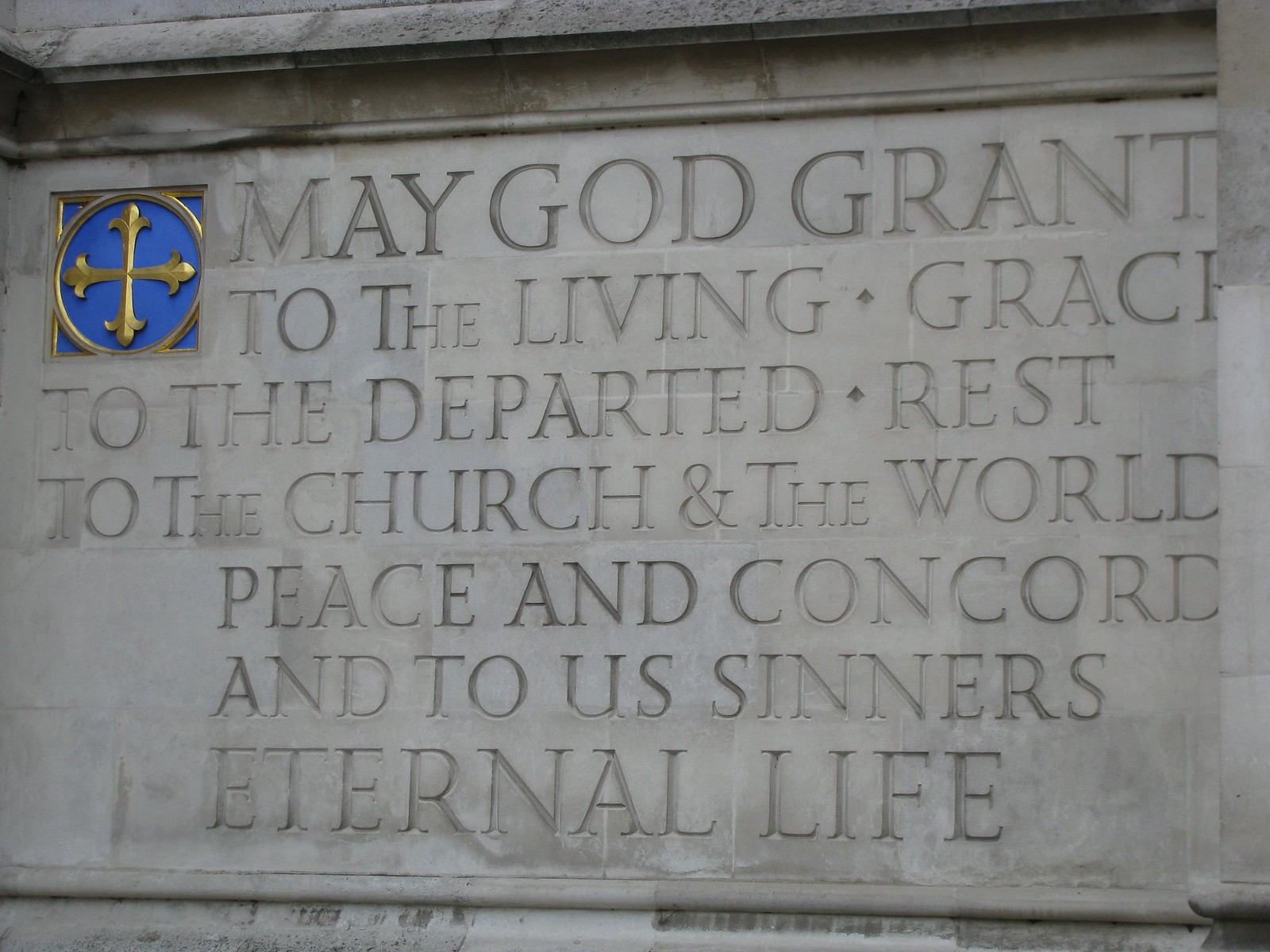This image features a weathered, gray stone plaque set against an outdoor concrete backdrop, likely at a church or religious location. The plaque takes up the entirety of the image and has an engraved inscription in all capital letters. In the top left corner, there is a blue background featuring a golden cross inside a golden circle, which is itself inside a golden square. The inscription reads: "May God grant to the living grace, to the departed rest, to the church and the world peace and concord, and to us sinners eternal life." The detailed composition and engraved message suggest a solemn and reflective setting.